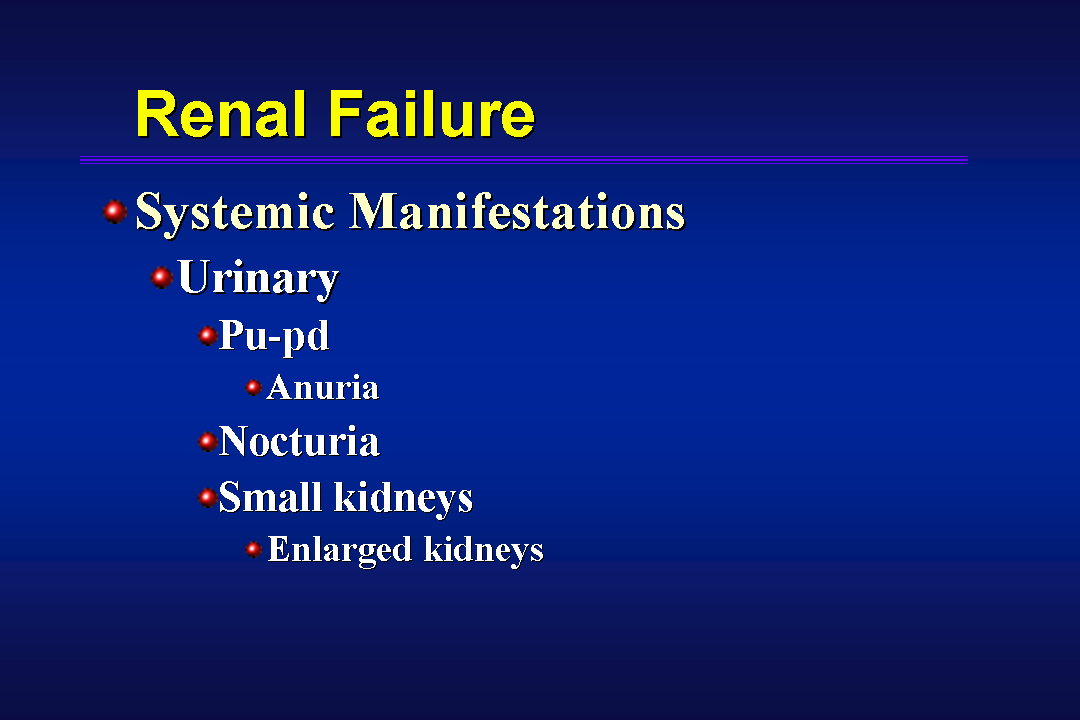The image displays a PowerPoint slide focused on "Renal Failure". The background features a gradient blue effect that transitions from a lighter blue in the center to a dark blue and almost black at the edges. At the top, the slide's title, "Renal Failure," is prominently displayed in yellow text. Beneath the title, a horizontal blue line spans the width of the slide. The slide includes several red bullet points, each associated with specific information: "Systematic Manifestations," "Urinary," "PU/PD," "Anuria," "Nocturia," "Small Kidneys," and "Large Kidneys." These bullet points appear sequentially from top to bottom, offering a detailed overview of the manifestations and conditions associated with renal failure.